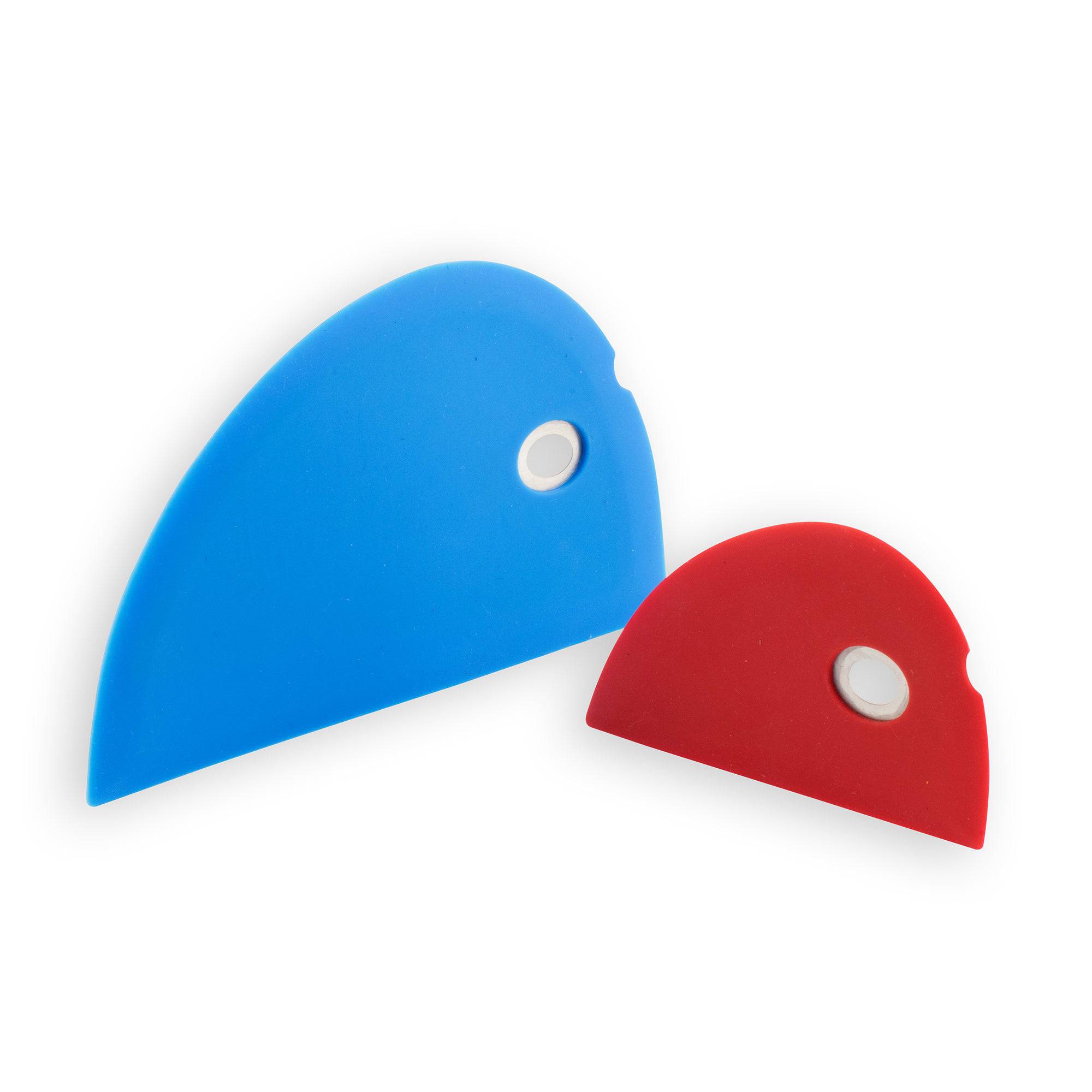The image features two semi-circular, plastic objects on a bright white background, giving the impression that they aren't casting any shadows. Both objects have flat bases and rounded tops, resembling arch shapes. The larger object on the left is a bright blue, while the smaller one on the right is red. Each object has a concave cutout about three-quarters of the way around, with a white circular feature positioned halfway up on the right side of the cutout. The design suggests an abstract depiction of a whale emerging from water, with the white circles and concave cutouts resembling eyes and mouths. The precise purpose of these objects remains unclear, although they could be interpreted as kitchen scrapers or abstract lenses.